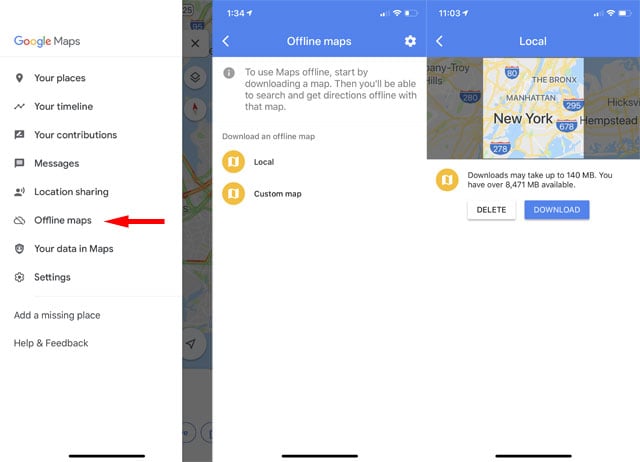The image showcases a screenshot of the Google Maps website. On the left side, there is a white background with a search bar at the top labeled "Google Maps." Below the search bar is a vertical menu featuring several options: "Your Places," "Your Timeline," "Your Contributions," "Messages," "Location Sharing," "Offline Maps" (highlighted with a red left-pointing arrow), "Your Data in Maps," "Settings," "Add a Missing Place," and "Help and Feedback." At the bottom of this section, there is a short horizontal black line.

To the right, there is a partially grayed-out section overlaid on a map. At the top of this section, a blue banner extends from the left to the right, displaying "134," along with icons for cell signal, Wi-Fi signal, and battery status. Below this, a left arrow and text reading "Offline Maps" appear, followed by another blue banner showing "1103," with icons for cell signal, Wi-Fi signal, and battery status again displayed.

Below the banners, a left arrow labeled "Local" is centered. The text on the left side instructs users on how to use maps offline by downloading a map, which will allow them to search and get directions without an internet connection.

At the bottom, there is a larger map section labeled with "New York, the Bronx, Manhattan." It notes that the download may take up to 140 MB and mentions that 8,471 MB is available. Options to either delete or download the map are provided.